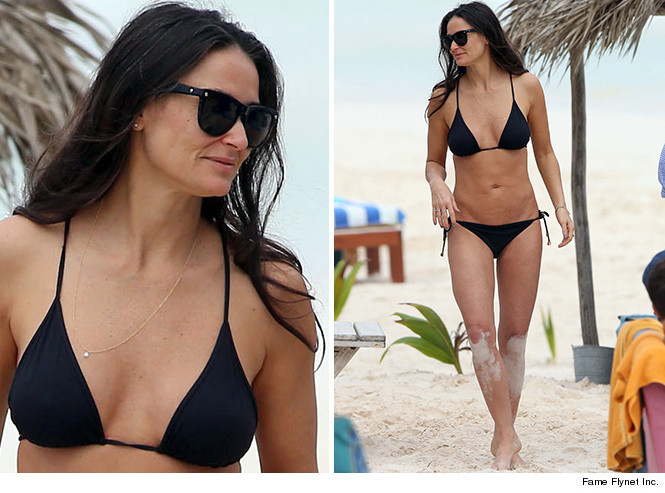The image is split into two parts, featuring the same middle-aged woman at the beach. In the left-hand side, there is a close-up view of her from her bosom to the top of her head. She has black hair, wears black sunglasses, a black bikini top, and a pendant. She is looking sideways and smiling, with her teeth visible. The background shows a clear sky and a glimpse of a tree. 

On the right-hand side, the full image of the woman is displayed. She is wearing the same black bikini two-piece and black sunglasses while walking through a beach setting. There is sand on her knees, suggesting she was kneeling. The background includes clear skies, plants, beach benches, and what might be a tiki hut roof. Another person is partially visible, cropped on the right. At the bottom of this side is a logo that reads "Fame Planet Ink dot". The overall setting appears to be midday at a resort beach.